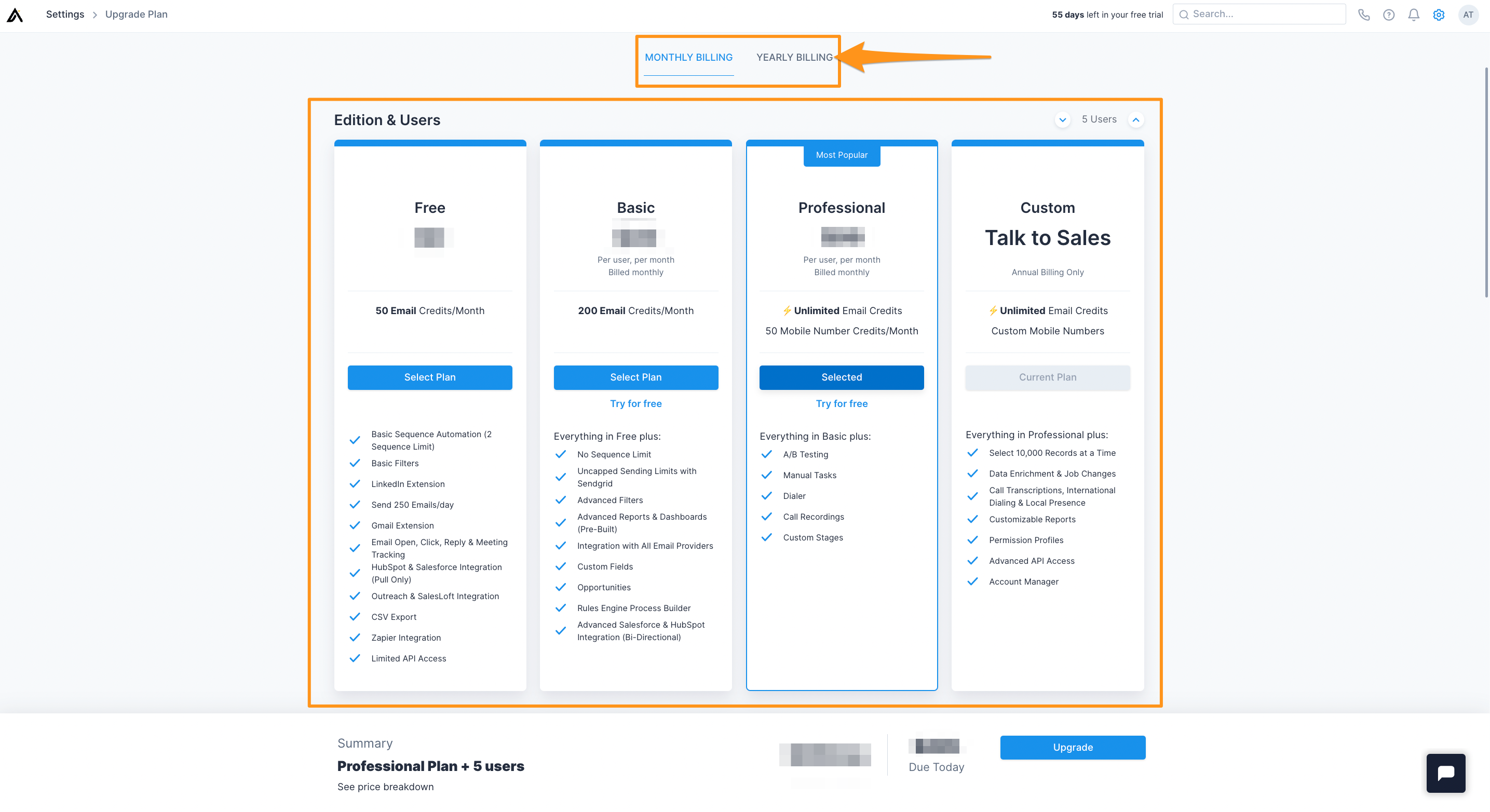The image displays a webpage showcasing subscription-based services. The central background of the page is a light gray color. In the upper left corner, a black logo is located next to the word "Settings," with "Upgrade Plan" positioned to the right. On the upper right side, there is a search bar, a phone icon, and additional icons.

In the upper center section of the page, a yellow or orange box highlights the "Monthly Billing" and "Yearly Billing" options, with an arrow pointing towards the "Yearly Billing" text. Below this area, another orange box presents various subscription plans: "Free Plan," "Basic Plan," "Professional Plan," and "Custom Talk-To-Sales Plan," each with detailed information beneath them. 

At the page's bottom, the "Professional Plan" option includes "+5 users," though the pricing information has been blurred out.